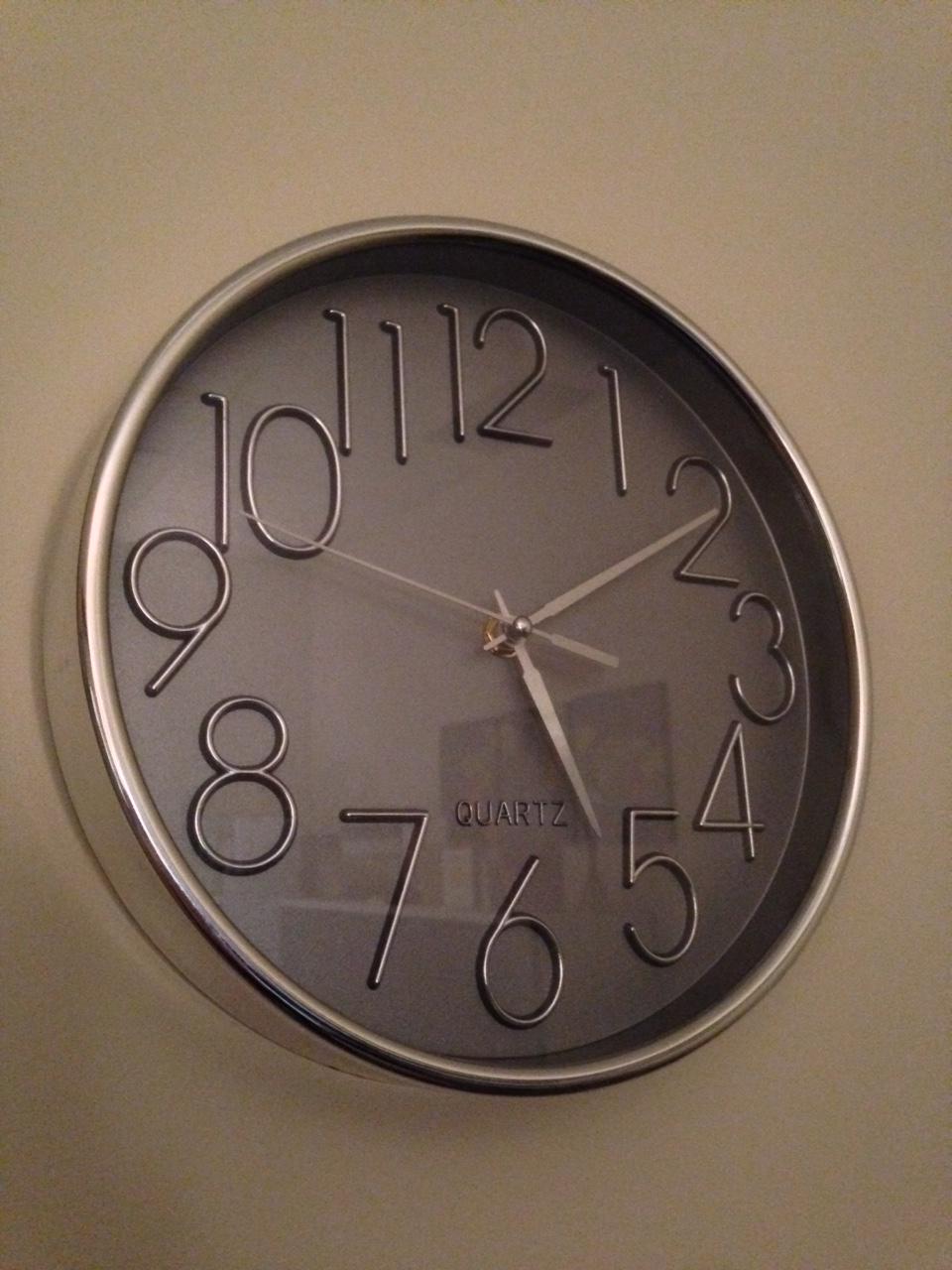This image features an elegantly designed clock mounted on a tan wall, presumably in an office setting. The clock, with its reflective surface, boasts a light silver outer rim and a darker silver inner face. The large, raised numbers are also silver but slightly darker, providing a striking contrast. The clock hands, equally silver, point to approximately 10 minutes past five, with the second hand positioned on the 10. The word "Quartz" is inscribed on the clock face, indicating its mechanism. Reflections on the clock's surface reveal additional details from the surroundings, including what appears to be a desk or credenza, possibly adorned with a statue resembling the Eiffel Tower, and a wall hanging or painting. These reflections are particularly prominent around the lower part of the clock, encompassing the 4, 5, 6, and 7 o'clock areas.